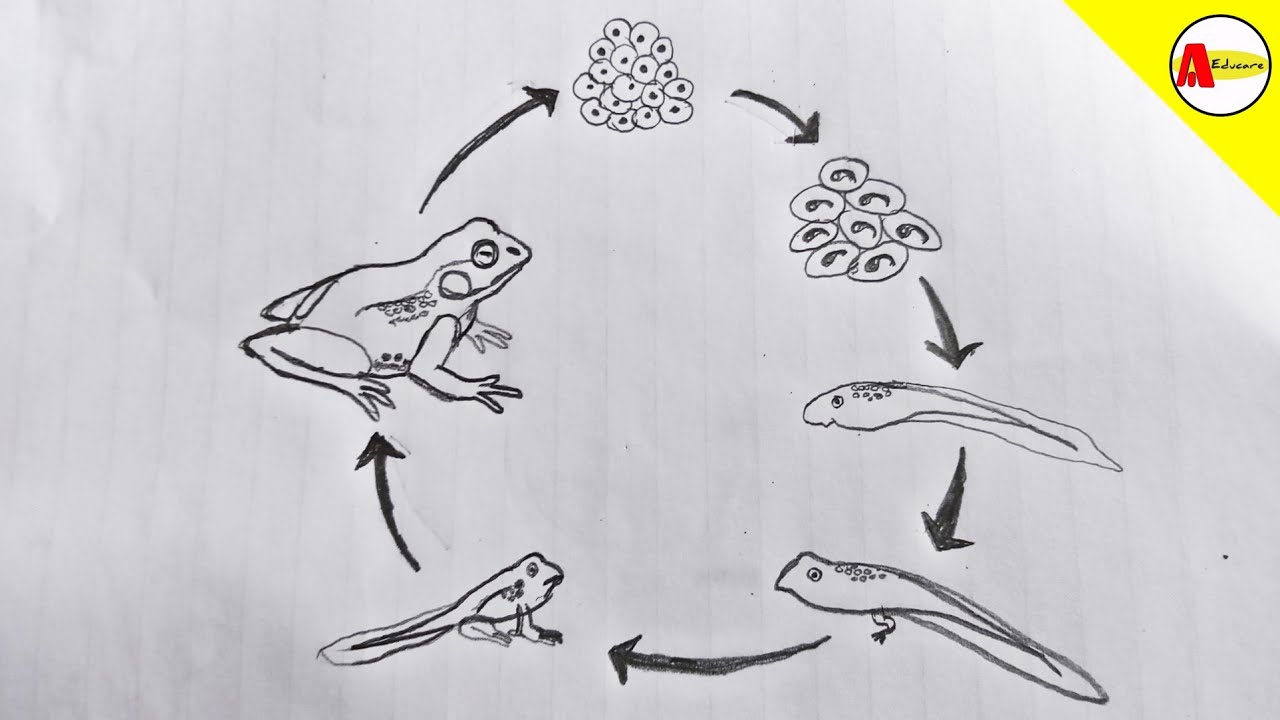This image features a meticulously detailed black and white sketch illustrating the life cycle of a frog. The drawing, executed on a horizontally-laid piece of lined paper turned to its blank side, reveals faint vertical lines in the background. At the top of the circular diagram, approximately at the 12 o'clock position, are a dozen or so frog eggs, depicted with black outlines and interior dots. A curved arrow directs the viewer clockwise to eight more eggs, each containing emerging tadpoles, then downward to the right to a single, white-outlined tadpole showing eyes and a tail. 

The cycle continues clockwise with another arrow pointing to an intermediate tadpole starting to grow hind legs, followed by another stage where the tadpole has both front and rear legs and retains its tail, now transitioning to resemble a frog. This stage is depicted around the 6 o’clock position. Another arrow then leads up to the 9 o’clock position, where a nearly mature frog, with four legs and a tail bump suggesting its metamorphosis, is illustrated. Finally, the diagram culminates with a fully developed frog at around the left side of the paper, facing right and slightly sitting up, with large protruding eyes and folded limbs, completing the life cycle. Each stage is clearly connected by curved arrows, emphasizing the continuous and cyclical nature of the process.